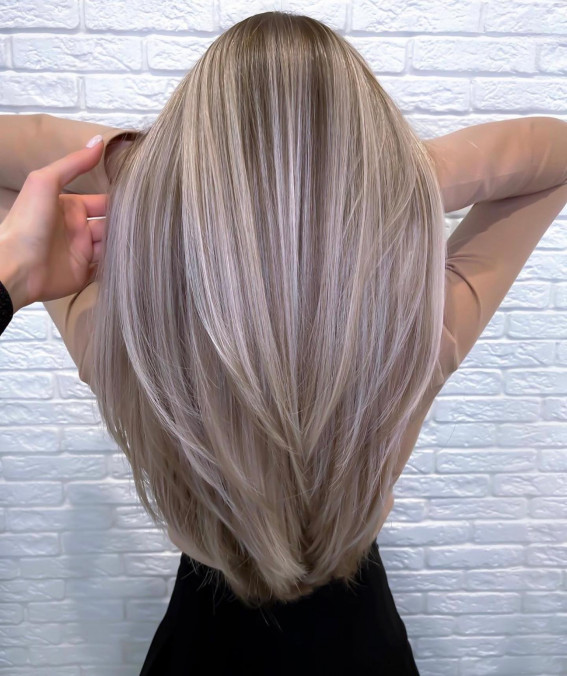A striking photograph features a woman with frosted blonde hair standing against a gleaming white brick wall. Her back faces the camera, highlighting the long, rich volume of her hair, interwoven with subtle gray and silver streaks, appearing healthy and undamaged. She is dressed in black, accentuated by a tan top peeking through. Her arms are raised, forming a triangle beneath her cascading hair. Another woman's delicate hand, adorned with white nail polish and partially covered by a black sleeve, is visible in the frame, suggesting an intimate interaction. The high resolution of the image captures every detail, from the woman's intricate hairstyle to the nuanced shadows on the wall, making it a visually captivating composition.